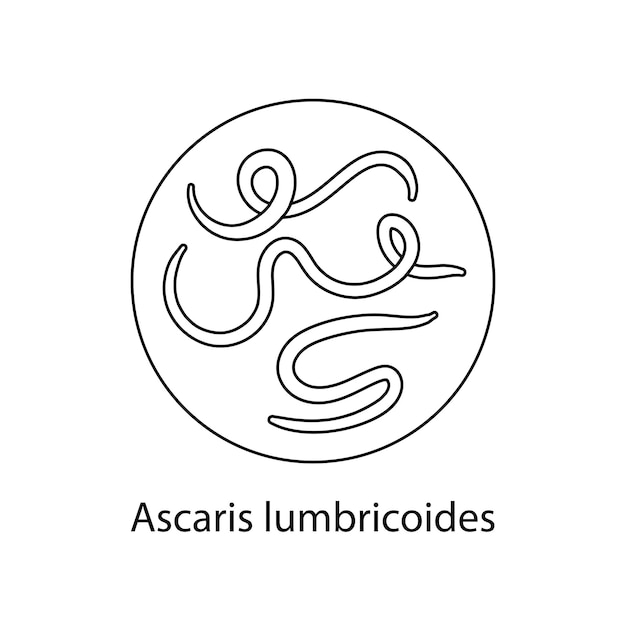This detailed black and white line drawing depicts a circle, resembling a petri dish, outlined by a thick black ring against a plain white background. Inside this circle are three distinct worm-like creatures, each outlined in black with a white interior. The first worm features a loop in its center, starting from its tail, looping up, and ending at its head. The second worm is elongated, with a loop positioned on its left side. The third worm is shaped like an 'S'. Below the circle, the Latin name "Ascaris lumbricoides" is inscribed, identifying these as parasitic worms that can infect humans and dogs. The scientific nature of the image suggests it might be a close-up view of the parasites under a microscope, likely sourced from a health textbook or website.